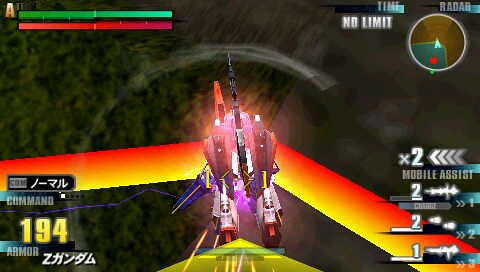The image is a screenshot from a video game. It depicts a futuristic scene viewed from behind a character who appears to be equipped with a robotic outfit and holding a narrow blue laser beam gun in their left hand. The character's back is glowing with red and yellow beams, as if emanating from a jetpack, suggesting they are in mid-air, perhaps having just jumped from an aircraft, with treetops visible far below. 

On the top left of the screen, a green and red bar is visible alongside a white circle containing brown and green segments, with white letters reading "No Limit" next to it. The top right corner shows the word "Radar." Beneath the left side of the screen, the text "Command" followed by "194" in yellow, "Armor," and some Asian characters are displayed. A square beam with orange and yellow hues intersects this area. 

In the center, there is a prominently featured futuristic apparatus, described as pink, yellow, and white, potentially part of the character's gear or weaponry. On the right side, the screen includes silver and white text "x2" with four arrows pointing left. Below this, the numbers 2, 2, and 1 are visible, indicating different types of available guns. At the bottom right, the phrase "Mobile Assist" is displayed.